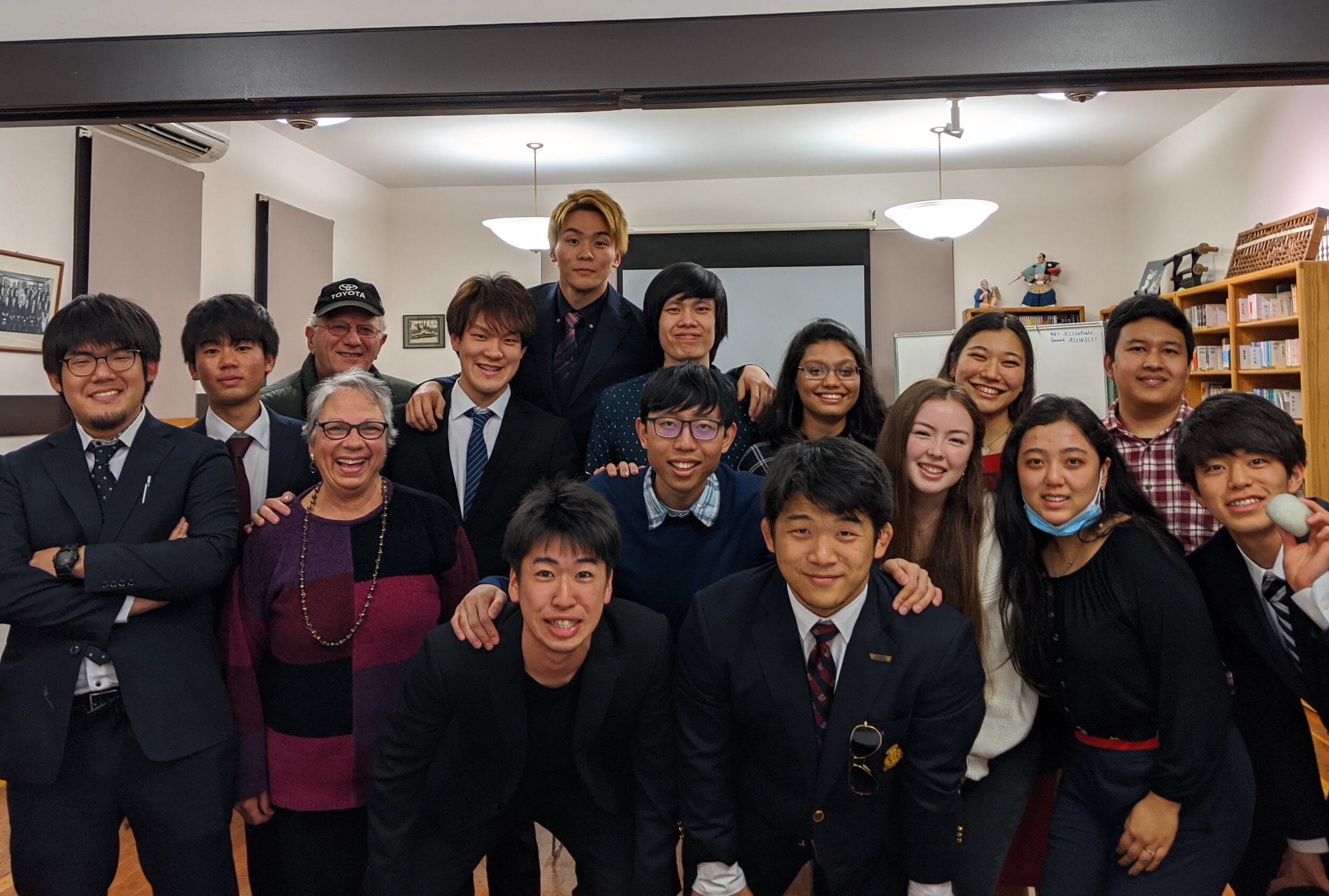This photograph captures a lively classroom scene filled with students predominantly of Asian ethnicity, estimated to be around 16 or 17 years old. They are all smiling and looking directly at the camera. The classroom backdrop features bookcases overflowing with books, bright lights suspended from the ceiling, and a noticeable poster board. The students, a mix of boys and girls, are dressed variably: the boys mostly in suits, some in casual attire like checkered shirts and jackets with caps, while the girls wear less formal outfits including jeans and various colored shirts, such as purple and white. Among the group are two older Caucasian adults, possibly in their 60s— a man in a blue ball cap standing behind a woman in a multi-purple checkered sweater adorned with a large bead necklace. The setting has the feel of a library, with bookshelves lining the walls and a glimpse of a doorway in the background.